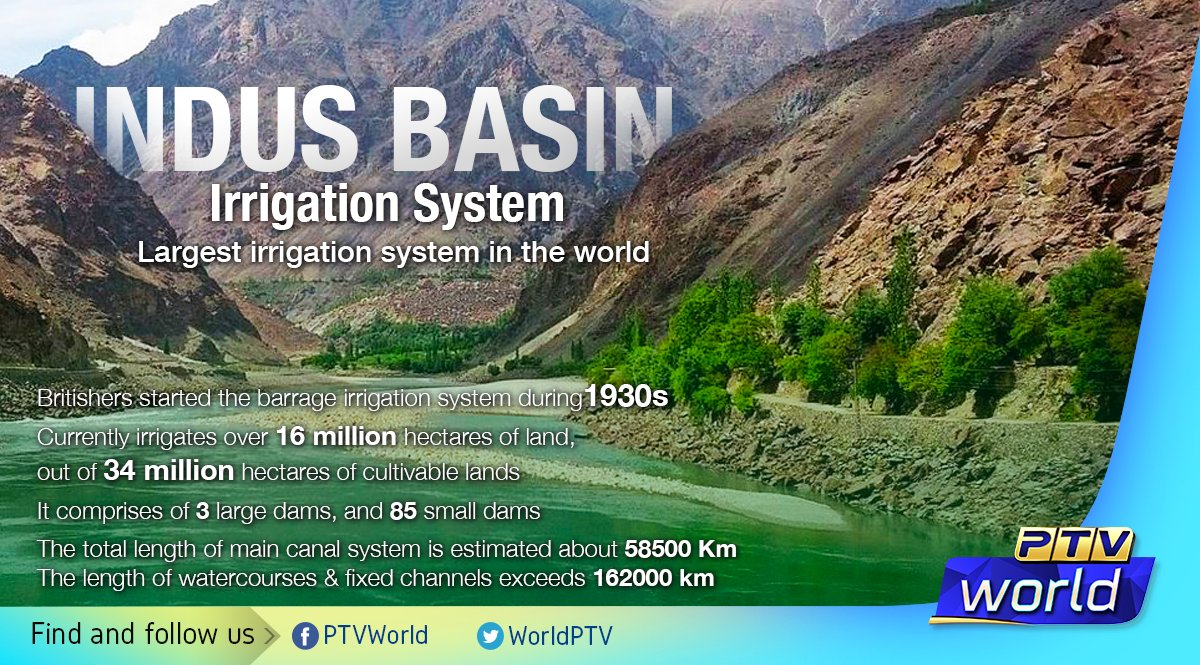The image depicts a promotional screen that showcases a picturesque scene of the Indus Basin Irrigation System, described as the largest irrigation system in the world. The centerpiece of the image is a greenish river flowing through a mountainous valley with imposing brown, rocky cliffs on either side. Adjacent to the riverbank, especially on the right, are signs of verdant life with clusters of green trees and bushes. Additionally, some smaller rocks and retaining walls can be seen near the water. 

In the foreground, bold white text provides detailed information about the Indus Basin Irrigation System: "Largest irrigation system in the world. Established by the British in the 1930s, it currently irrigates over 60 million hectares of land out of 34 million hectares of cultivable lands. It includes three large dams and 85 smaller dams, with the main canal system extending approximately 58,500 kilometers and the total length of watercourses and fixed channels exceeding 162,000 kilometers."

A blue and yellow footer spans the bottom of the image, inviting viewers to "find and follow us" on social media, specifically on Facebook under PTV World and on Twitter under World PTV. The lower right corner of the image features the PTV World logo, indicating the source of this promotional ad. In the lower-left corner, the label "PTV World" reaffirms the broadcaster's identity.